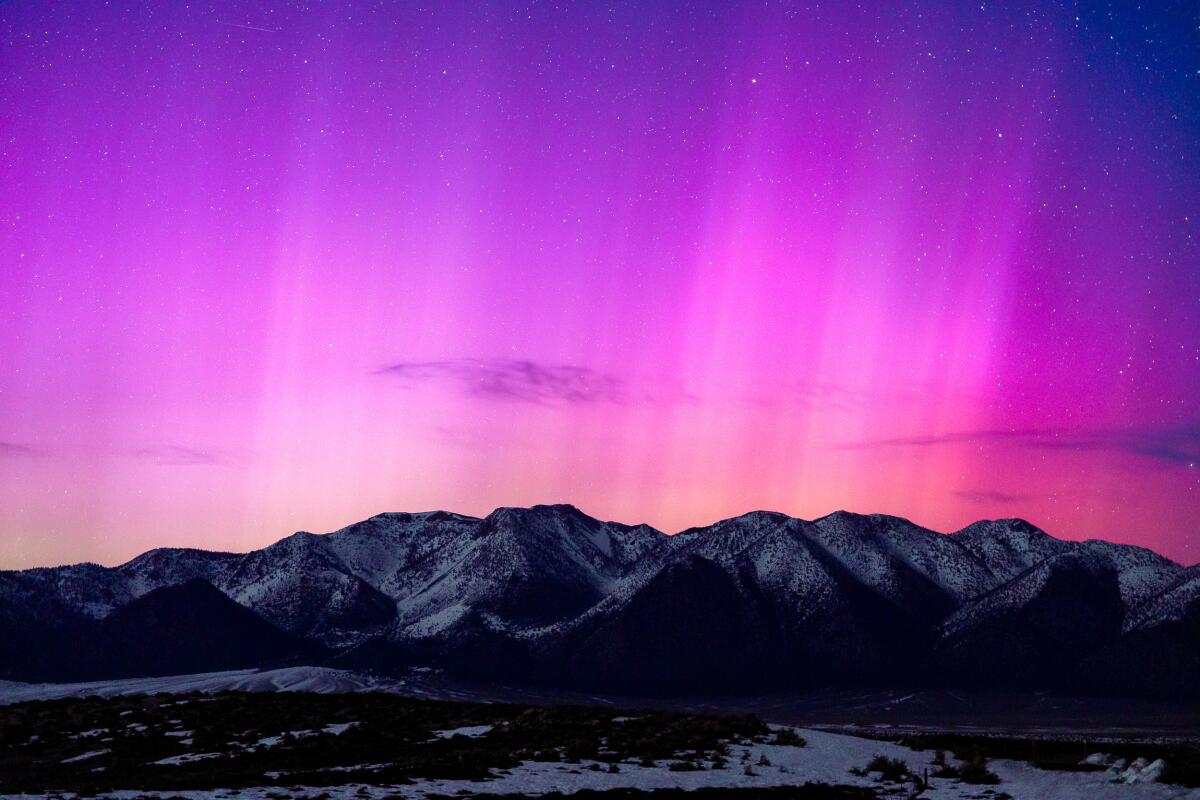This image captures a breathtaking outdoor scene at dusk, showcasing a mesmerizing aurora borealis display in the night sky. The phenomenon predominantly features a radiant pink glow that transitions into deep purples and light peach hues in the center, illuminating the vast expanse above. The sky is dotted with a scattering of stars and a few wispy clouds.

In the foreground, a snow-capped mountain range spans the lower third of the picture, its dark silhouette contrasting sharply with the luminescent sky. The mountainous terrain is cloaked with patches of snow, extending to the snowy ground below. Subtle beams of light from the aurora emerge behind the mountains, creating an ethereal display that stretches upward, bathing the entire scene in a surreal glow.

The foreground also reveals tufts of snow-covered grass, adding texture to the wintry landscape. The overall effect is a stunning portrayal of nature's light show against a serene, starlit sky, making for a visually compelling and intricate composition.